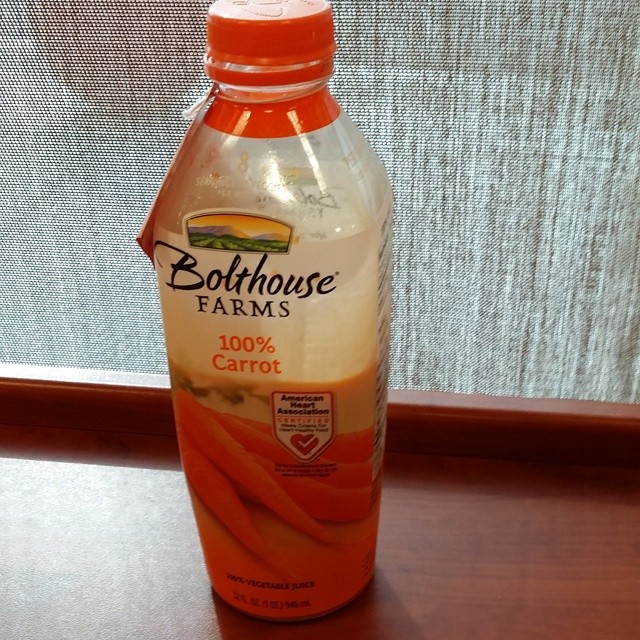The image depicts a half-full Bolthouse Farms smoothie drink placed slightly left of center on a reddish-stained wood table or windowsill. The plastic bottle is topped with an orange cap and features a vibrant design with a colorful illustration of a farm, mountains, and a blue sky backdrop, highlighting the brand's natural and wholesome imagery. Prominently, the label displays “Bolthouse Farms” in bold black cursive lettering, followed by “100% Carrot” in orange text, and an image of five carrots. The American Heart Association's certified logo, a red heart with a check mark, is also visible. The background is a drab khaki screen, semi-translucent, letting some light through and revealing an outdoor space, possibly a deck with a red ball in the top right corner.